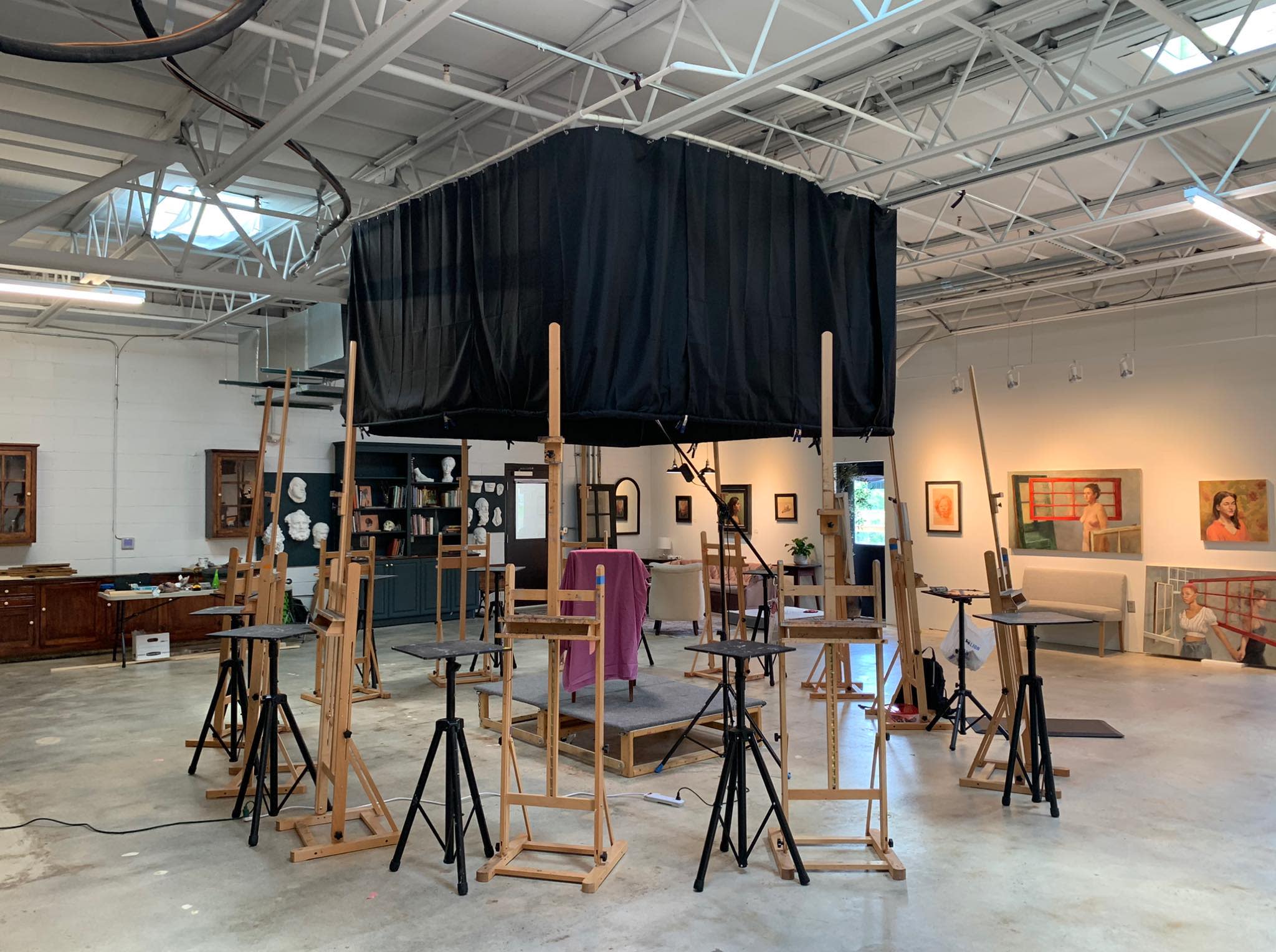This detailed, full-color photograph captures the interior of an art studio with artificial lighting. The square-shaped image reveals white walls adorned with various artworks including paintings and sculptures. The ceiling, crisscrossed with metallic girders that likely provide structural support, features multiple lights concentrated in the upper corners, casting spotlights on the exhibited artwork. The floor is a shade of white, enhancing the room's minimalist aesthetic. 

Central to the composition is a large black canvas mounted on what appears to be a wooden easel, drawing immediate attention. Surrounding the main easel are other simple wooden stands and table easels, positioned strategically for individual artistic workspaces. Despite being well-equipped for creativity, the room is void of any people, evoking a calm, almost anticipatory atmosphere. 

In addition, there are various tables and racks arranged in a circular manner around the room, adding to the studio's functional layout. Notably, the space includes two doors located at the back center, further defining the room's entry and exit points. The colors throughout the image range from blacks and browns to brighter hues like orange, purple, fuchsia, green, and several metallic shades, contributing to a vibrant yet professional ambiance. Overall, the photograph skillfully encapsulates the essence of an art studio in ready anticipation of its artists.